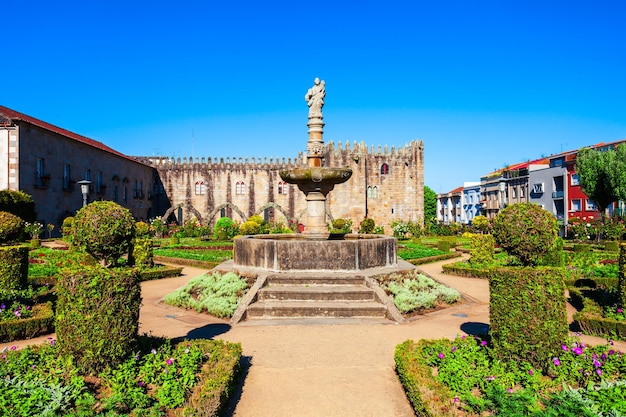The image depicts an antiquated courtyard dominated by a weathered, inactive fountain at its heart. This stone fountain, set upon a circular platform reachable by three distinct steps, features a mysterious statue, possibly of a man, though the details are obscured. Radial garden pathways converge at this central point, framed by meticulously sculpted bushes and sporadic flowers that denote a vibrant season, likely spring. To the rear, an aged castle stands as a testament to history, its walls showing signs of deterioration. Adjacent to the right of this historic structure are a series of modern, colorful apartment buildings, each about two stories high, painted in shades of red, gray, beige, and pale blue. Above, the sky is a deep blue gradient, adding to the serene yet juxtaposed setting of old and new architectural elements.